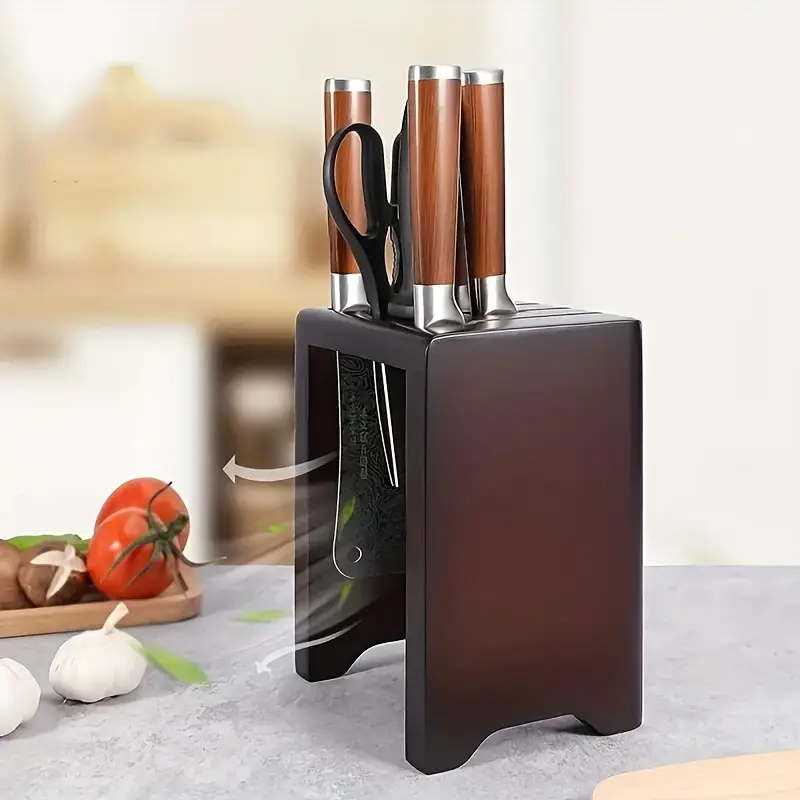The image depicts a detailed product shot of a sophisticated knife set, prominently featuring an innovative holder. This holder, resembling an upright black box or a finely crafted dark wood arch with a reddish hue, securely houses a collection of culinary tools. Within the holder, there are three knives, including a meat cleaver and another that could serve as a steak knife, along with a practical pair of scissors. Each utensil is neatly positioned in vertical slots that prevent them from slipping through, thanks to widened handles.

Surrounding the knife holder, the scene is set with a concrete tabletop adorned with fresh culinary elements, including tomatoes, garlic cloves, and a variety of vegetables. The background hints at a blurred kitchen scene, enhancing the authentic culinary atmosphere.

Graphical elements, such as arrows and airflow streaks, are superimposed over the image, suggesting an airflow mechanism within the holder designed to keep the knives dry or sterile. These artistic renderings add a futuristic touch to the practical design, underlining its functionality. The scene, with its combination of detailed product and creative graphics, effectively communicates the innovation and utility of the knife holder, making it a compelling advertisement.